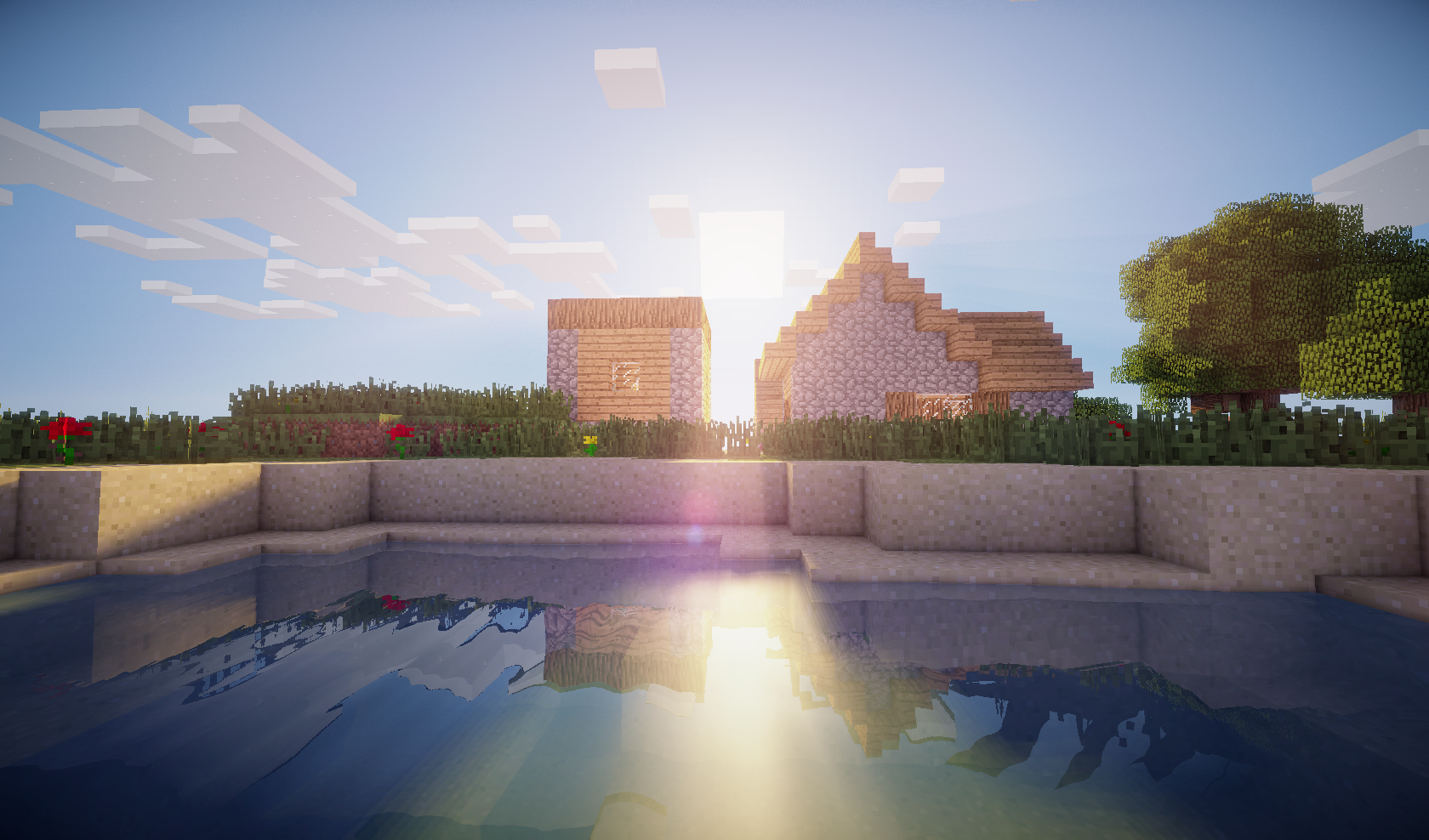A vibrant screenshot from the game Minecraft captures a sunny day in a meticulously crafted landscape. In the azure blue sky, variously shaped formations hover, resembling clouds but constructed from in-game materials. The scene is dominated by an intricate arrangement of brick buildings with wooden accents, complemented by patches of lush green grass. Concrete walls border the area, framing a large, serene pool with a bluish tint reflecting the clear sky. The absence of any characters focuses attention on the architectural beauty and peaceful ambiance, highlighted by the blue, tan, and brown hues of the buildings and the contrasting colors of the natural elements. The overall palette includes vivid blue for the sky, white clouds, and bright green grass, perfectly capturing a tranquil moment in this Minecraft creation.